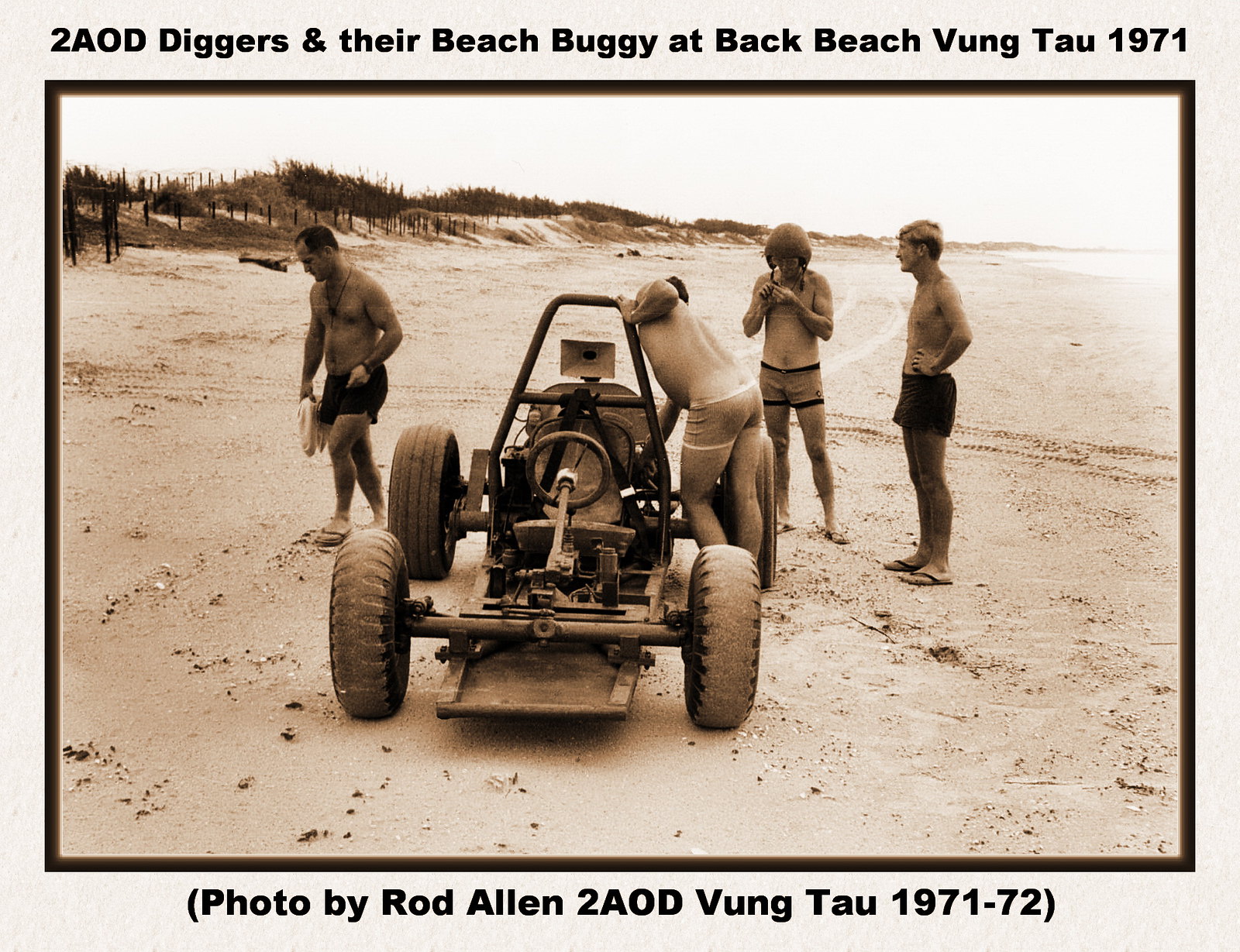This sepia-toned photograph, bordered with a textured white frame on a black background, captures a scene at Back Beach, Vung Tau in 1971. The photo, credited to Rod Allen, features four men—three on the right and one on the left—all dressed in swimsuits. Central to the image is a beach buggy or dune buggy, positioned on the sandy shore with its front facing the viewer. The vast beach environment extends into the background with visible sand dunes, a fence, and some bushes on the left. The bright sky reflects off a sliver of water seen in the upper right corner. The man on the left appears to be walking away, possibly carrying some material, while another is leaning down to inspect the buggy. The immersive outdoor ambiance of the photograph is accentuated by the serene yet dynamic composition of people and machine against the expansive sandy beach. The caption inscribed at the top reads, "Two AOD diggers and their beach buggy at Back Beach, Vung Tau, 1971," and at the bottom, "Photo by Rod Allen, two AOD, Vung Tau, 1971-72."